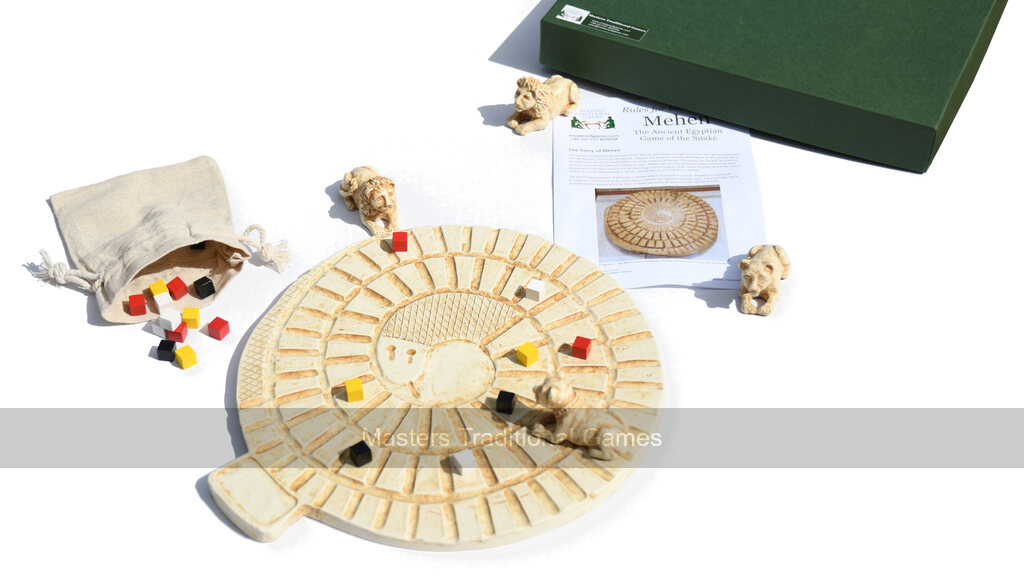This image captures a board game designed to resemble an ancient, traditional game called "Master's Traditional Games." The board is circular with a spiral design that evokes the appearance of a rattlesnake coiling inward, culminating at the center. The entire setup is rendered in an ivory or bone color, but it might actually be made from plastic crafted to look like aged stone. Notably, the game board has a small handle-like protrusion on the bottom left side for carrying.

The board is inhabited by eight multi-colored game pieces in red, black, white, and yellow hues. Arranged on and around the board are four exquisitely hand-carved lions—two male and two female. Two lions are positioned on the board at the 11 and 1 o'clock positions, while the other two lions lie beside the handle. The entire scene is set against a whitish-gray background, enhancing the ancient, monochromatic aesthetic of the game.